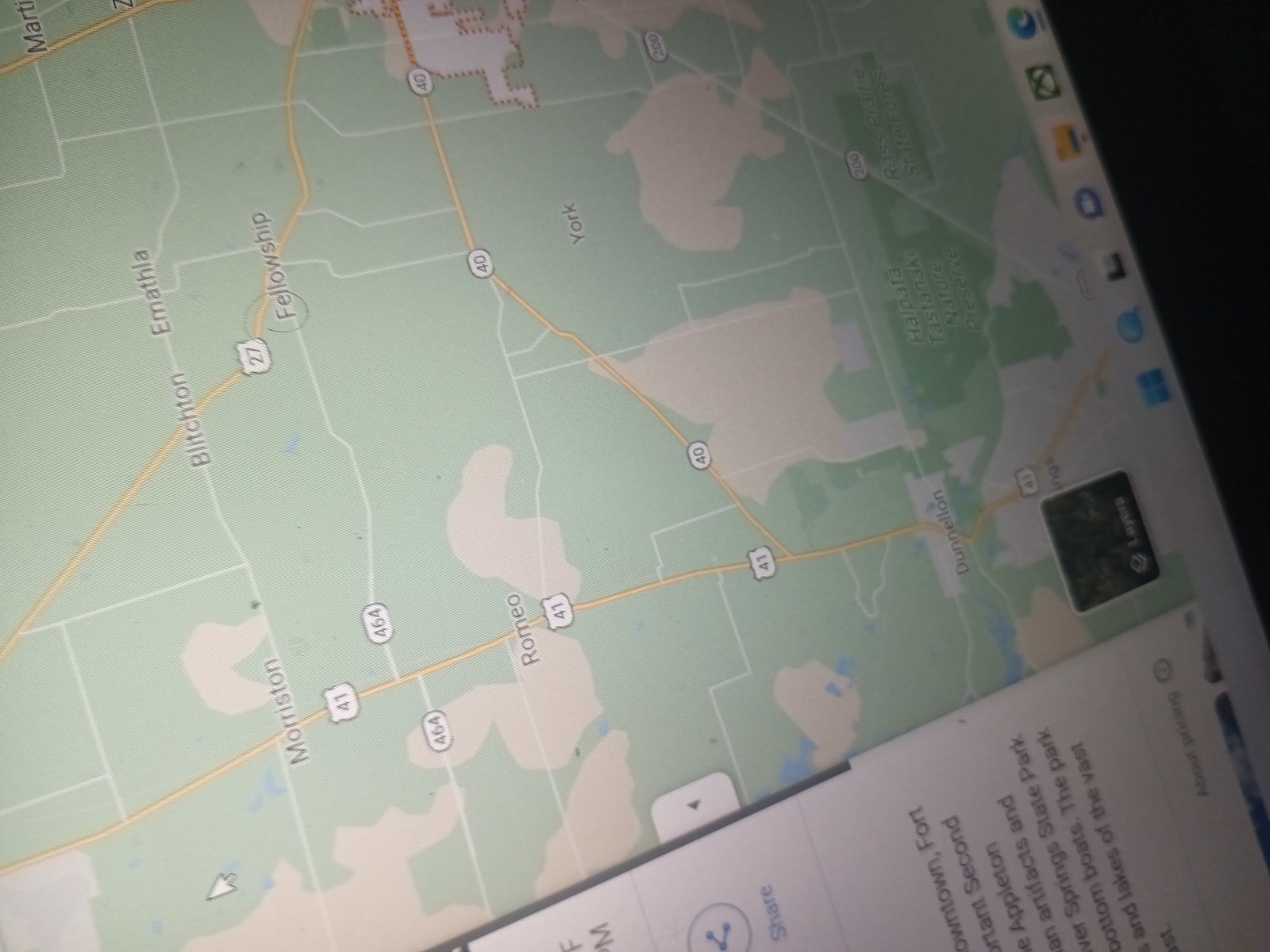The photograph captures a sideways-oriented computer screen displaying a detailed map. The hallmark of a computer interface is apparent with the white mouse cursor, shaped like an arrow, visibly present on the map. The screen's bottom edge, which appears on the right side due to the tilted orientation, features a grey taskbar housing various icons including the Windows logo, a Search icon, a Messenger or Zoom logo, the Microsoft Edge logo, and the Xbox logo. The map itself is depicted in a palette of green, yellow, white, and tan.

Prominent roads are highlighted in distinct colors: Route 41 is marked in yellow, Route 464 is illustrated by a white line, and Route 27 runs diagonally in yellow in the upper left corner. Another yellow line designates Route 40, which stretches from Route 41 to the edge of the map. Key locations identified on the map include Morriston, Romeo, Blichton, Amethyla, Fellowship, and York.